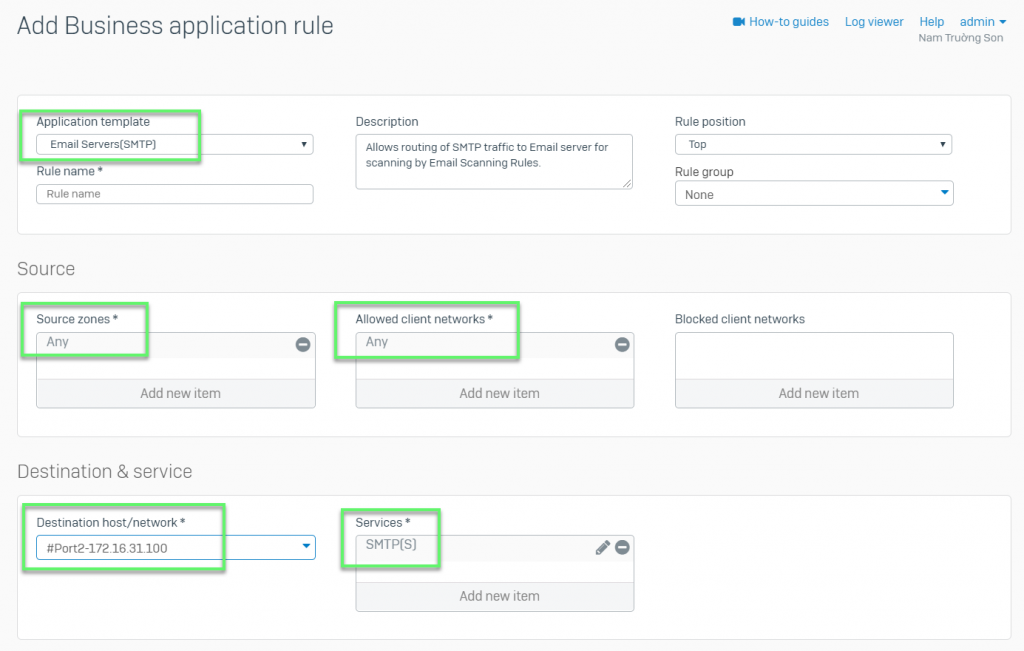This cropped screenshot provides a focused tutorial on completing a specific panel within an application interface. At the top, the title "Add Business Application Rule" is prominently displayed in black letters. To the right, there are four clickable blue hyperlinks: "How to Guides," "Log Viewer," "Help," and "Admin." The "Admin" section includes a dropdown menu. On the far right, the name "Narn Truong Son" appears in small, light grey letters.

The interface features three large, white, rectangular panels. 

In the first panel at the top, several highlighted areas in green boxes direct attention to specific fields. The "Application Template" field, highlighted in green, is set to "Email Servers (SMTP)." Below, fields for "Rule Name," "Description," "Rule Position," and "Rule Group" are arranged from left to right.

The middle panel begins with the "Source" category, marked in large letters at the top left. Directly below, "Source Zones" is highlighted in a green box, set to "Any." To the right, the "Allowed Client Networks" field, also highlighted, is set to "Any."

In the third panel, the "Destination and Service" category starts with "Destination Host Network" on the left, highlighted in green. Adjacent to it on the right, the "Services" field is similarly highlighted to indicate necessary input areas.

This detailed screenshot serves as an instructional guide for users to accurately fill out the application panel fields, ensuring correct configuration and input.